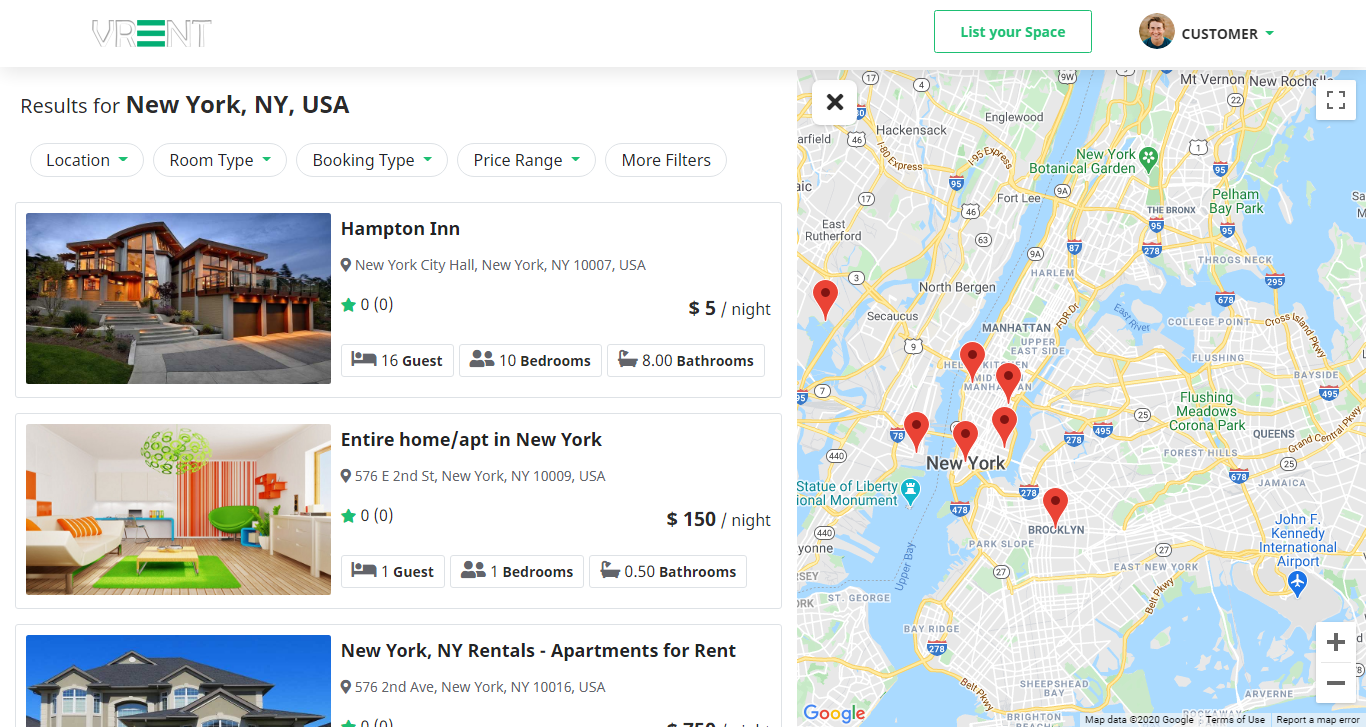In the upper left corner of the image, there is light text displaying "VR" followed by three small green horizontal lines and "NT". To the right, enclosed in a green rectangle, are the words "list your space". Moving further right, there is a circular icon featuring a smiling man's profile picture labeled "customer".

Below this, there is a map snapshot from Google Maps, predominantly showing white and blue hues representing land and water areas. Central to the map is "New York" indicated in black text, accompanied by numerous red markers highlighting various locations. To the left, the text reads "Results for New York, New York, USA".

The first listing is the "Hampton Inn", depicted as a brown building illuminated at night. The caption reads "Hampton Inn, New York City Hall, New York". Below this, an interior image showcases a room with green carpet and orange curtains, labeled "entire home apartment in New York $1.50 a night".

In the bottom left corner, an image shows a large beige building with a gray roof. Adjacent text reads "New York, New York rentals apartments for rent."